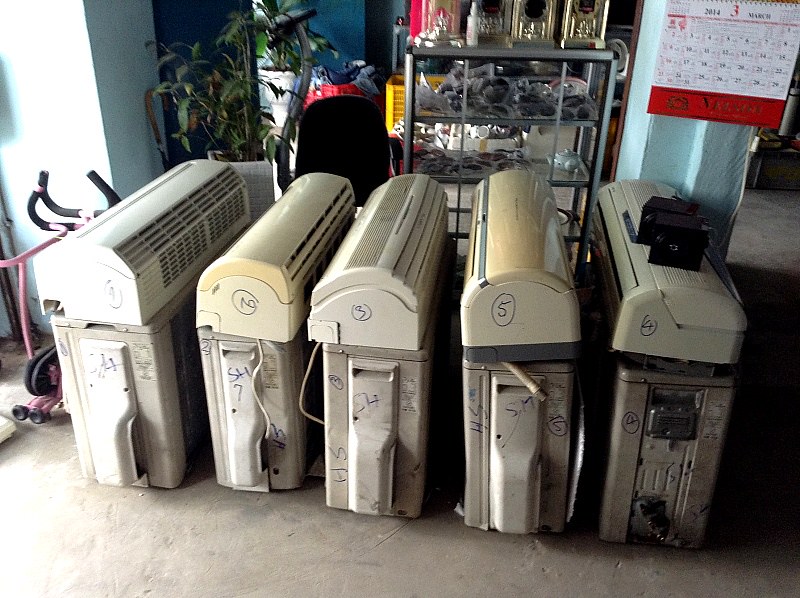The image depicts a row of five similar mechanical units, likely heating or air conditioning units, positioned on a concrete floor within a shop. Each unit has numbers written in black marker on their ends, with the sequence reading from left to right as four, six, three, five, and four again. The units feature a combination of plastic and metal, with rounded tops and directional vents. The unit on the far right has two or three small black rectangular boxes placed on top of it. Behind these units is a backdrop that includes a rack loaded with various items, a black office chair, and an aqua-colored post with a wall calendar hanging from it. The calendar is open to March 2014. A houseplant can be seen behind the unit to the far left. The floor appears to be concrete, and natural light floods the scene from the left side, likely through a window or door.